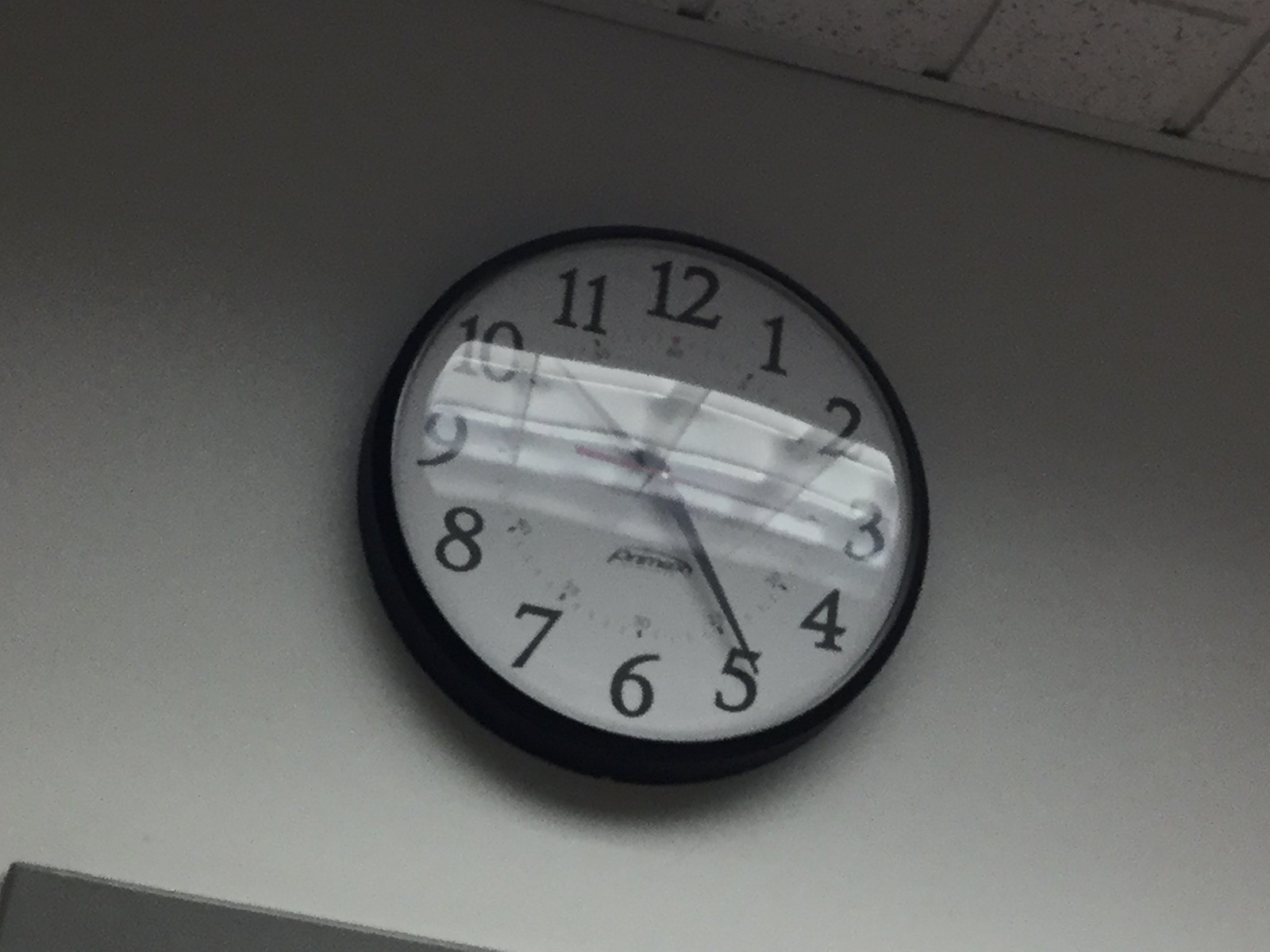This photograph captures a round, wall-mounted analog clock prominently displayed against a stark white wall. Suspended beneath a drop-down tile ceiling, the clock features a sleek black frame that contrasts sharply with its pristine white face. Black numerals from 1 to 12 are elegantly printed around the clock's perimeter, clearly marking the hours. The time-telling hands include two pointy, black needle-shaped hour and minute hands, accented by a bright red second hand that adds a pop of color to the monochrome scheme. The image is slightly blurred, obscuring the manufacturer's name printed at the center of the clock face, adding an air of intrigue to this everyday object.